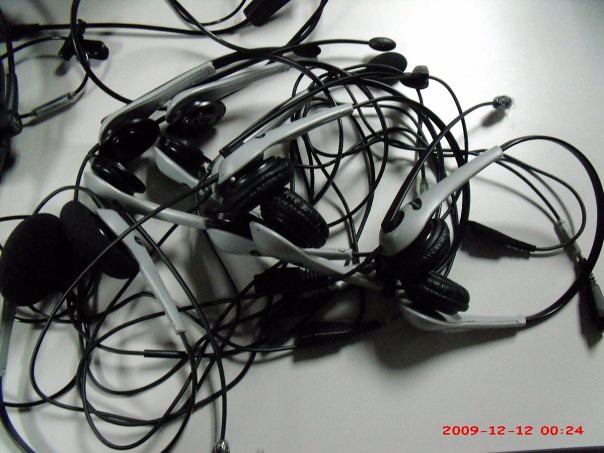This photograph, dated "2009-12-12 00:24" in red letters at the bottom corner, showcases an assortment of over-the-ear headsets haphazardly piled together on a white surface. The headsets, uniformly two-toned with gray earpieces and black cords, microphones, and headphone ports, lie tangled in a mish-mashed heap. The microphones are connected by wires that crisscross and twist together, adding to the chaotic arrangement. A light source from above casts shadows around the edges of the image, highlighting some additional cords in the top left corner.